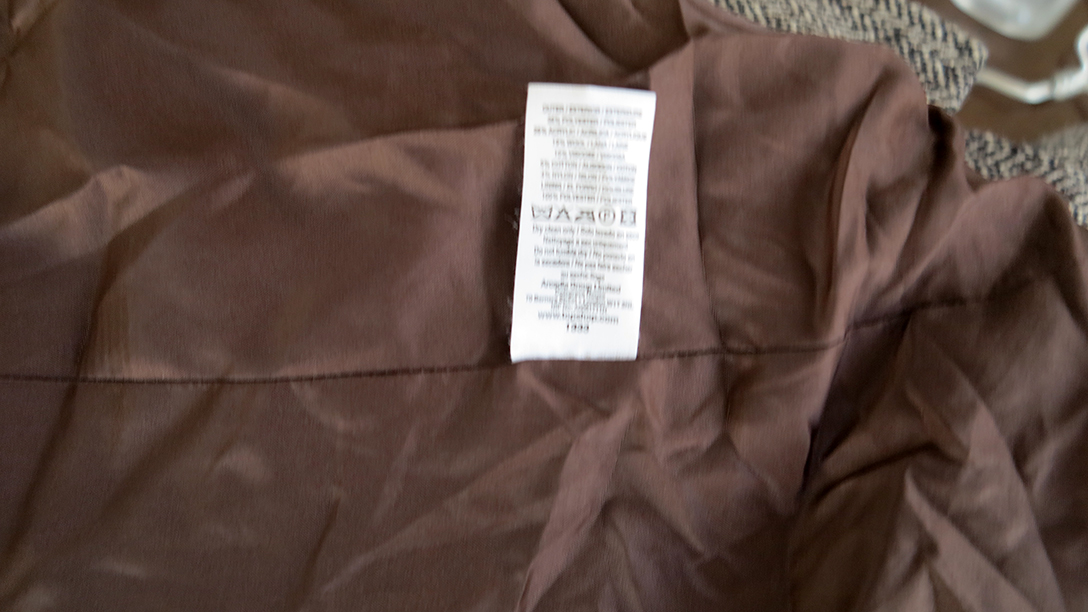A crumpled, brown cloth with a silky, smooth, and slightly shiny texture stretches across the image. At the center of the fabric is a long rectangular white tag adorned with black writing. The top right corner showcases a section of white fabric featuring black zigzag patterns, alongside a brown area and an ambiguous white pipe-like object. In the bottom left, the folds and shadows of the cloth form a vague skull-like shape, complete with discernible eye sockets and a nose. A single stitch line runs horizontally across the middle of the brown cloth, with no additional stitching visible elsewhere.